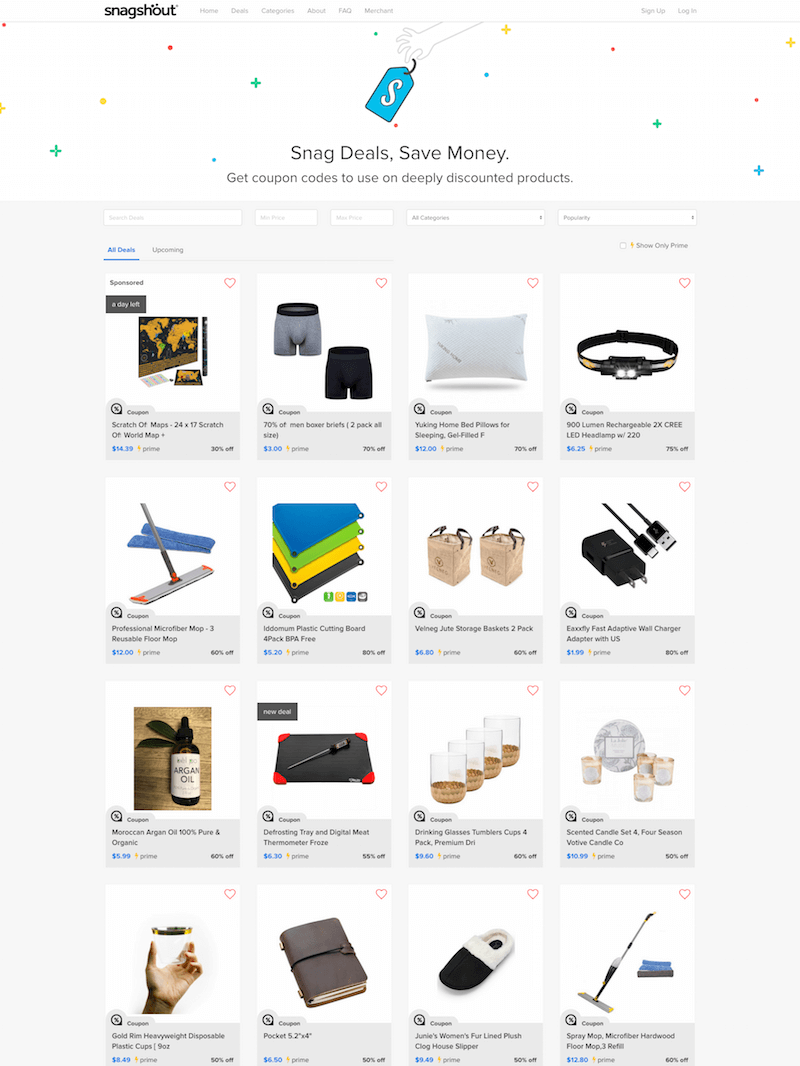A detailed caption for this image could be:

"The Snag Shout website features a visually engaging design with a unique umlaut above the 'H' and 'O' in 'Shout'. The top of the page is adorned with a gray navigation bar, though its small text is hard to discern. Below this, the main section of the website is displayed in a white field, highlighted by a colorful array of stars, figures, and dots in red, yellow, green, and blue. An illustrated right hand holds a blue tag, emphasizing the site’s cartoonish aesthetic. The tagline reads: 'Snag deals, save money, get coupon codes to use on deeply discounted products.' 

The lower section boasts a wide variety of products available for purchase. Key items include scratch-off maps, men's underwear, pillows, a battery-powered headlamp, mop heads with replacements, and more. Additional offerings include a variety of products such as green, yellow, and blue items with pull corners, bags, and different kinds of USB plug-ins. The assortment is extensive, promising something for everyone looking to snag a deal."